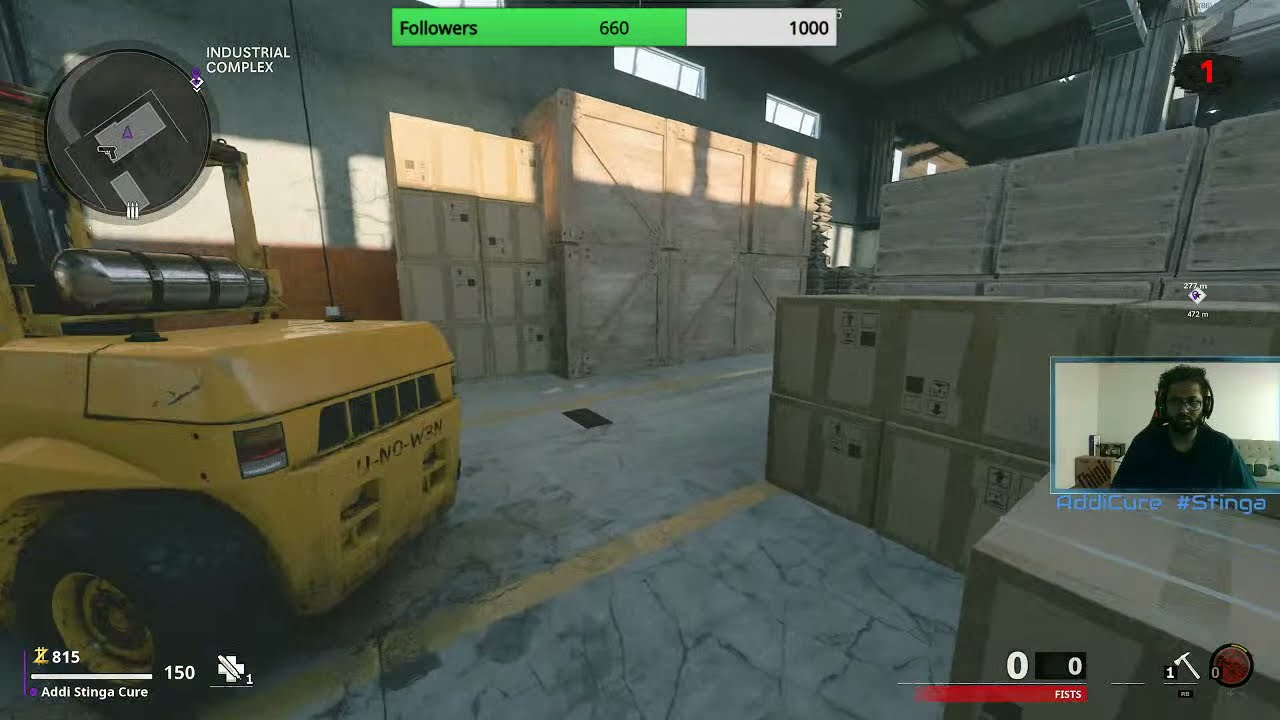This vertical rectangular image is a computer screenshot from a video game set in a warehouse environment. Dominating the left side of the scene is a large yellow construction vehicle, which has a steel canister mounted above where the windshield would be. The background is filled with stacked wooden crates reaching up to narrow windows positioned almost at ceiling height. The concrete floor features two yellow stripes, and additional boxes and wooden crates are seen on the right side of the image. 

In the lower-left corner, there are several white text elements: the number 815 with a line beneath it, and Addie, Stinga, Cure, number 150 accompanied by a small cross icon with a number one. Centered at the top of the screen, the word "followers" is highlighted in green with a count of 660 in black text beside it, followed by a gray background displaying the number 1000 in black. Near the construction vehicle, there's small white print indicating "industrial complex."

On the right-hand side of the screen, a rectangular inset shows the player, a man wearing a black t-shirt and headset, with glasses and a beard, seated in a room with white walls. Below his video feed, the text reads "Addie Cure, #Stinga."